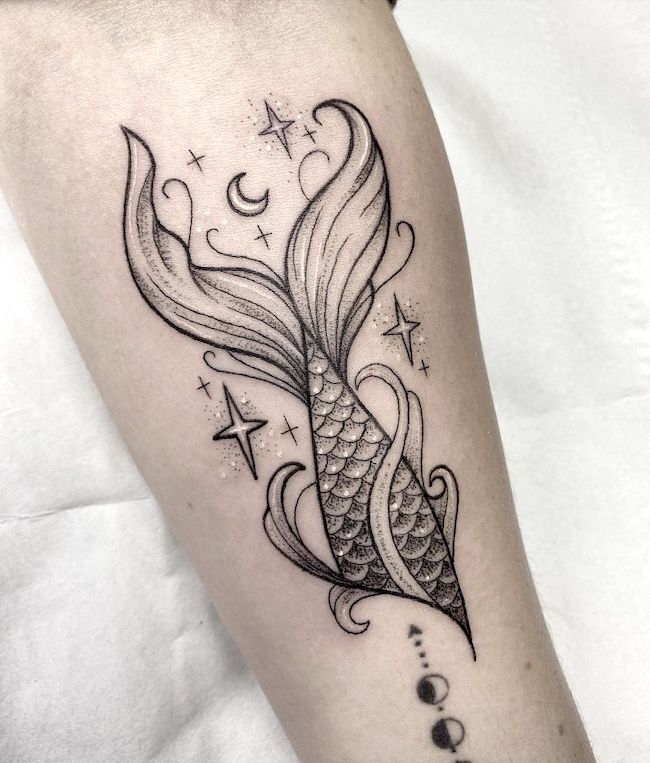This black and gray tattoo, located on a fair-skinned forearm, features an intricate, flowy depiction of a mermaid tail that spans from the middle of the forearm to the wrist. The tail appears to be emerging from within the arm, giving it a surreal, fantastical quality. The design includes white ink sparkles that add a majestic touch, enhancing the tail’s celestial appearance. Surrounding the mermaid tail are various geometric shapes and moon phases, including quarter and half moons, depicted with detailed shading. An arrow points towards the tail, adding directionality to the piece. The tattoo is set against a white cloth background, highlighting its black and white palette and emphasizing the arm's placement and the tattoo’s contrast against pale skin.